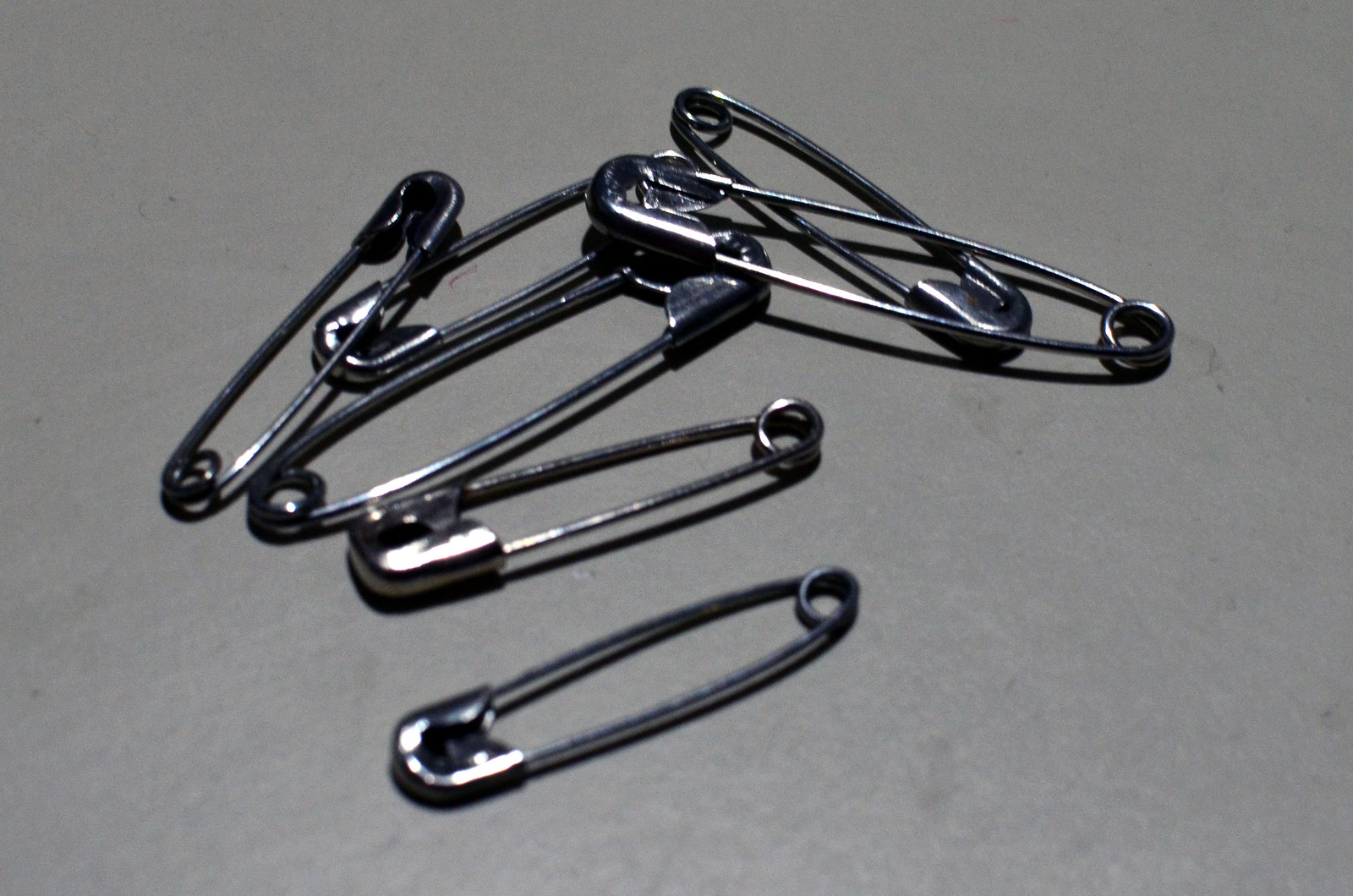This color photograph features seven silver safety pins arranged in a somewhat jumbled pile on a medium-tone gray background, which appears to be a sheet of paper with visible imperfections and flecks of fibers. The safety pins vary in size, with some being larger and others medium-sized, and they also differ in design based on the shape of their heads. All the pins are in the closed position. Four of the safety pins are aligned diagonally, starting nearly halfway in from the left side and extending to the middle of the bottom section, with three of these pins' heads pointing left or lower left and one pointing upper right. A fifth pin overlays this arrangement, with its head directed toward the center top and its tail slightly below the middle left side. There is another large safety pin positioned over the heads of the first two pins in the diagonal row, with its tail aimed right. Finally, a smaller safety pin lies beneath this large one, with its tail near the top center and pointing toward the middle right. The photograph is wider than it is tall.